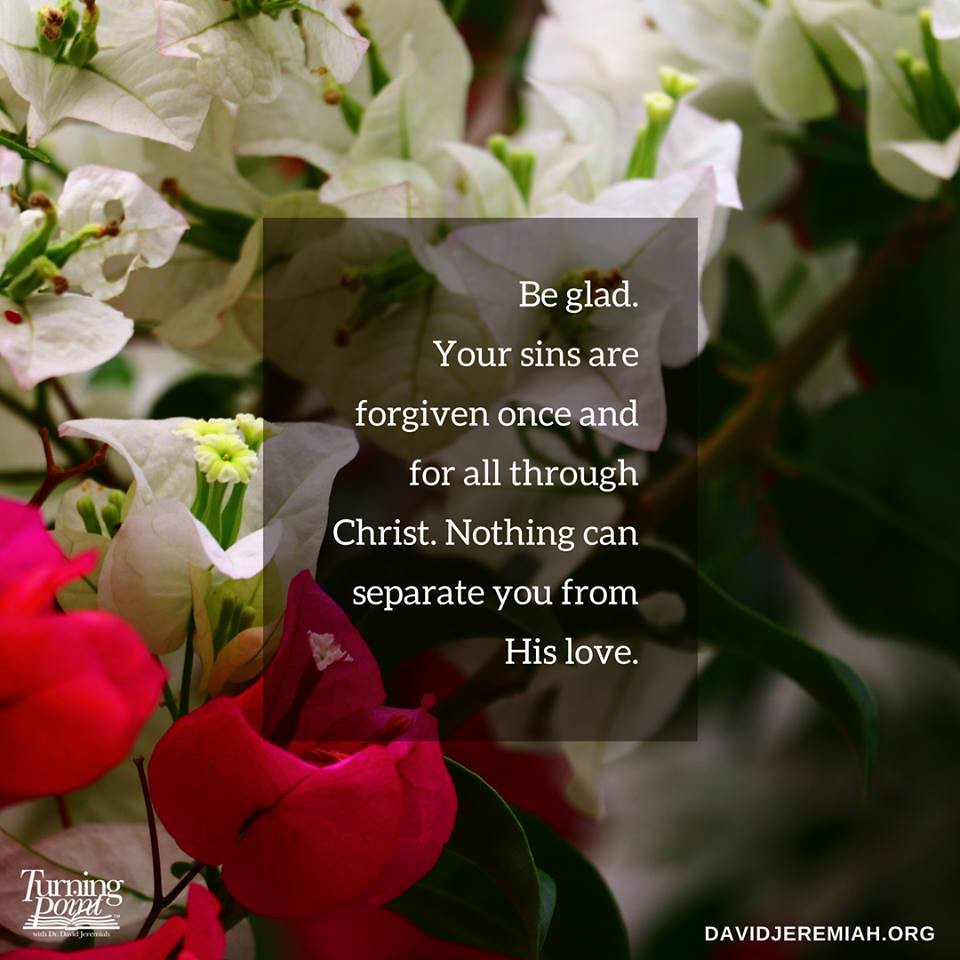The image is a detailed photograph of a garden showcasing a variety of flowers, including vibrant red roses and white tulips. The central focus of the image is a message overlayed in an opaque gray rectangle with white font. The text reads: "Be glad. Your sins are forgiven once and for all through Christ. Nothing can separate you from His love." This religious message, indicative of a greeting card or inspirational poster, is complemented by additional text at the bottom of the image: "Turning Point" in the bottom left and "DavidJeremiah.org" in lowercase on the bottom right. The light source in the image appears to come from the top left, illuminating the flowers in that area and casting a subtle shadow on the bottom right. The right side of the image is slightly blurry, adding a soft focus effect.